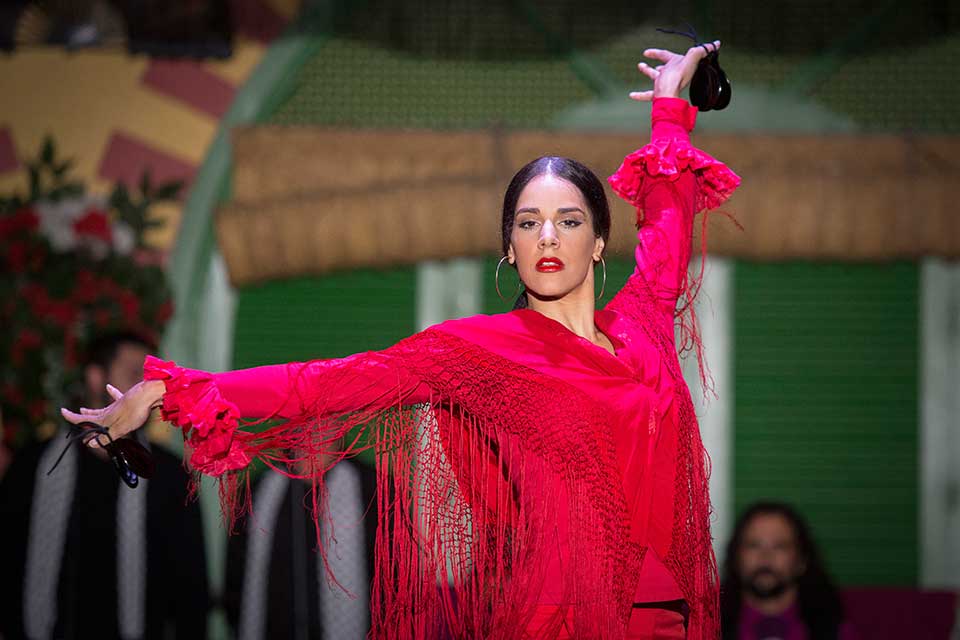This detailed, photorealistic image captures a flamenco dancer, striking a dramatic pose. The dancer, a Spanish-looking woman with dark, tied-back hair and large hoop earrings, has a serious expression. She wears bright red lipstick and a vibrant, almost neon pink-rose red blouse, accentuated with ruffles at the cuffs and fringes hanging down from her arms. Her right arm is outstretched, holding a pair of black castanets between her thumb and forefinger, with fingers gracefully turned up. Her left arm is raised above her head, also holding castanets, and her fingers elegantly splayed. The photograph is cropped at her hips, so the lower part of her attire is not visible, though a hint of a skirt can be seen.

The background, slightly out of focus, reveals an arch-like doorway on a yellow building with green accents, possibly shutters or louvers. Two men, seemingly dressed in dark robes with white clerical collars, stand fuzzily in the backdrop. Another man with long hair, a mustache, and a trimmed beard, wearing a red collared shirt, is seated on the right side of the photo. The scene evokes a sense of traditional Spanish culture and intrigue.